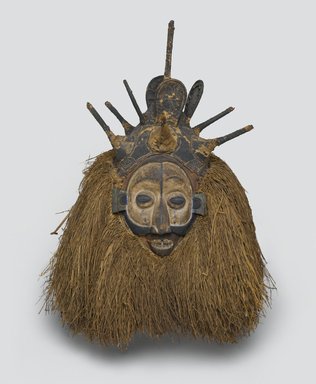This photograph features a museum-quality tribal mask, likely originating from Africa or New Guinea. The centerpiece of the composition is a carved wooden mask with expressive features, including two rounded eyes, a triangular nose, and a small mouth crafted on a separate wooden segment. The mask is brown and black in color and is topped with an intricate headdress. This headdress consists of a crown with six upward-pointing spikes, three on each side, and a central round projection culminating in a seventh spike.

Attached to the edges and the back of the mask is a lavish decoration made from long, thin, grass-like fibers. These fibers, resembling dried straw or husk, envelop the mask, extending downward and outward. They possess a rich gradient, coming in shades of dark honey to dark beige. The entire piece is displayed against a plain white background, which accentuates its intricate craftsmanship and the natural materials used, creating a striking and detailed example of tribal art, suitable for museum display.